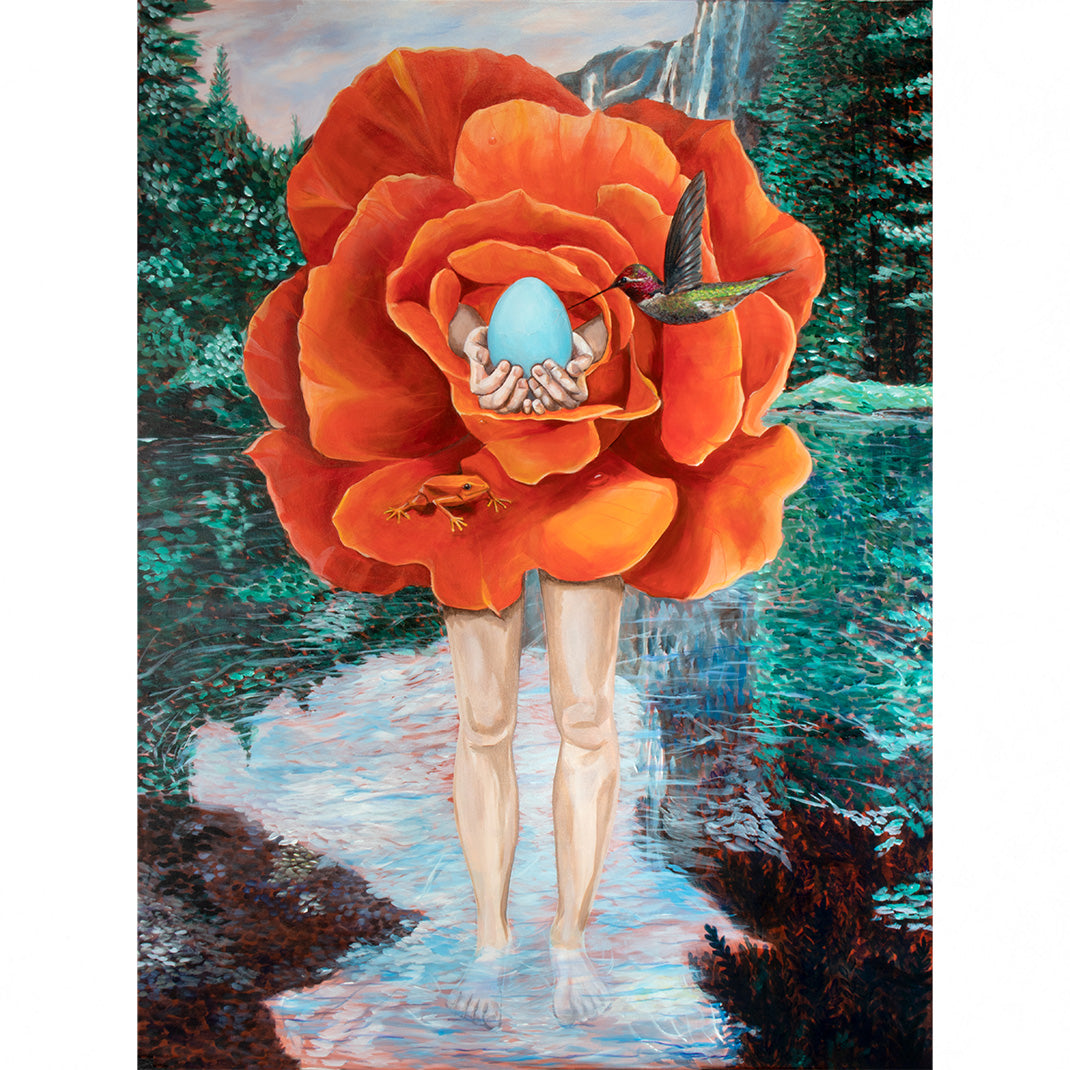In this detailed and vibrant abstract artwork, the focus is on a surreal figure whose lower body consists of bare legs submerged in bright blue water up to the ankles. The torso transforms into a giant orange and red flower, blending seamlessly with the human legs. Emerging from the center of this flower are two bare forearms and hands cupping a light blue egg. To the right of the egg, a hummingbird with a greenish-yellow belly, red head, and black wing extends its long beak to touch the egg. An orange frog perches inconspicuously on one of the lower petals of the flower. Surrounding this figure, the water teems with green and red plants, particularly visible in the bottom corners of the image. The background features a dichotomy of scenery: to the left and right, vibrant green leaves and trees, including evergreens, and in the distance a grayish sky with tall cliffs or mountains. Pink veins run through the bright green and turquoise ground, adding to the fantastical environment. The entire scene is depicted in bold and unusual colors, creating a dreamlike outdoor setting bathed in daylight.